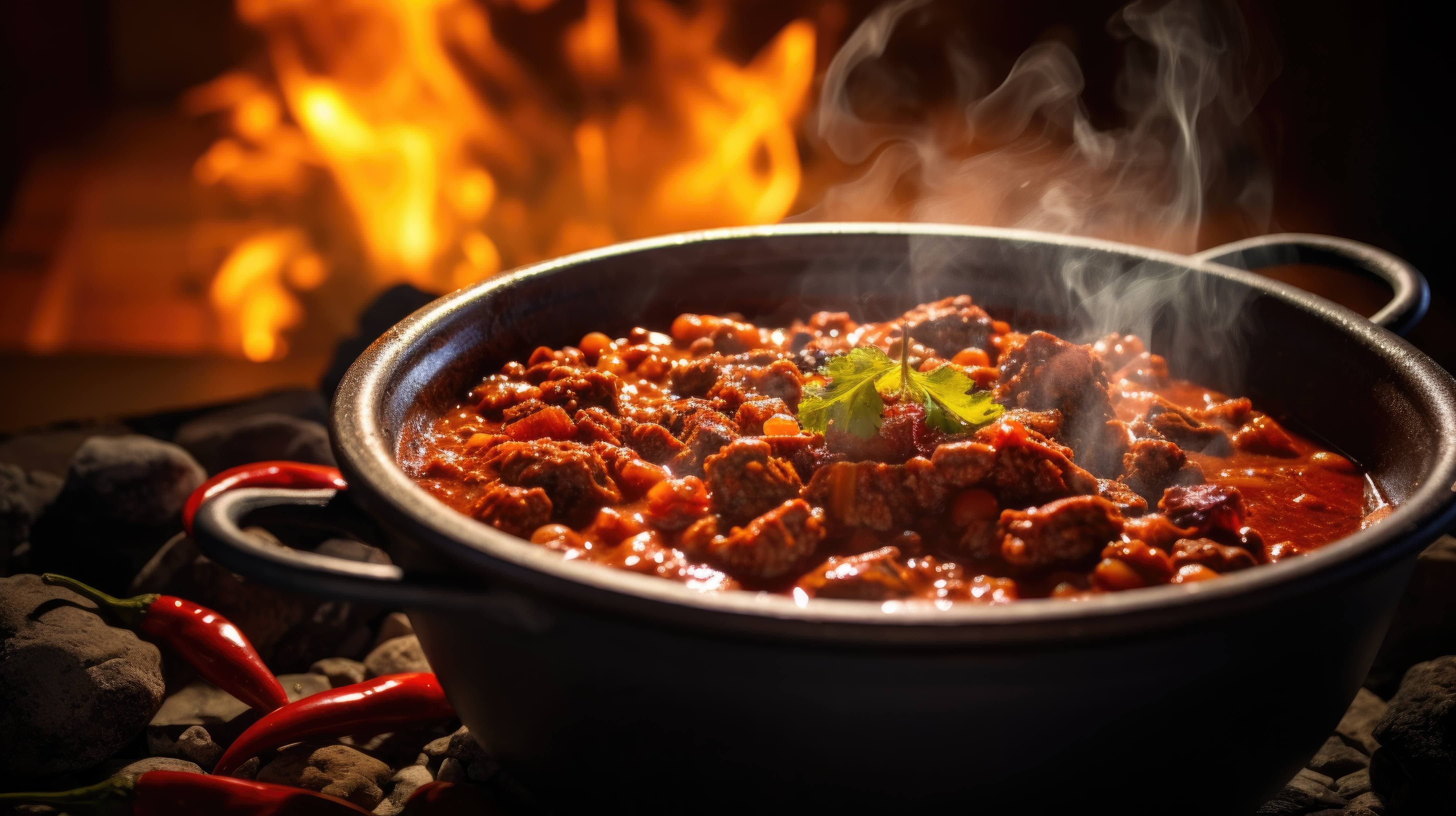A richly detailed image captures a rustic culinary scene centered around a cast iron bowl brimming with savory, reddish-brown chili. Wisps of fragrant steam rise tantalizingly from the hearty dish, accentuating its warmth. On top of the chili, chunks of succulent meat are visible, adding texture and depth to the dish. Crowning the ensemble is an upside-down sprig of cilantro, or a similar green herb, providing a fresh pop of color. Surrounding the bowl, a scattering of small, elongated red chilies with pointed tips add both a visual and spicy kick to the tableau. In the softly blurred background, a comforting fire glows, casting its light warmly over the scene and hinting at a cozy, dimly lit setting.